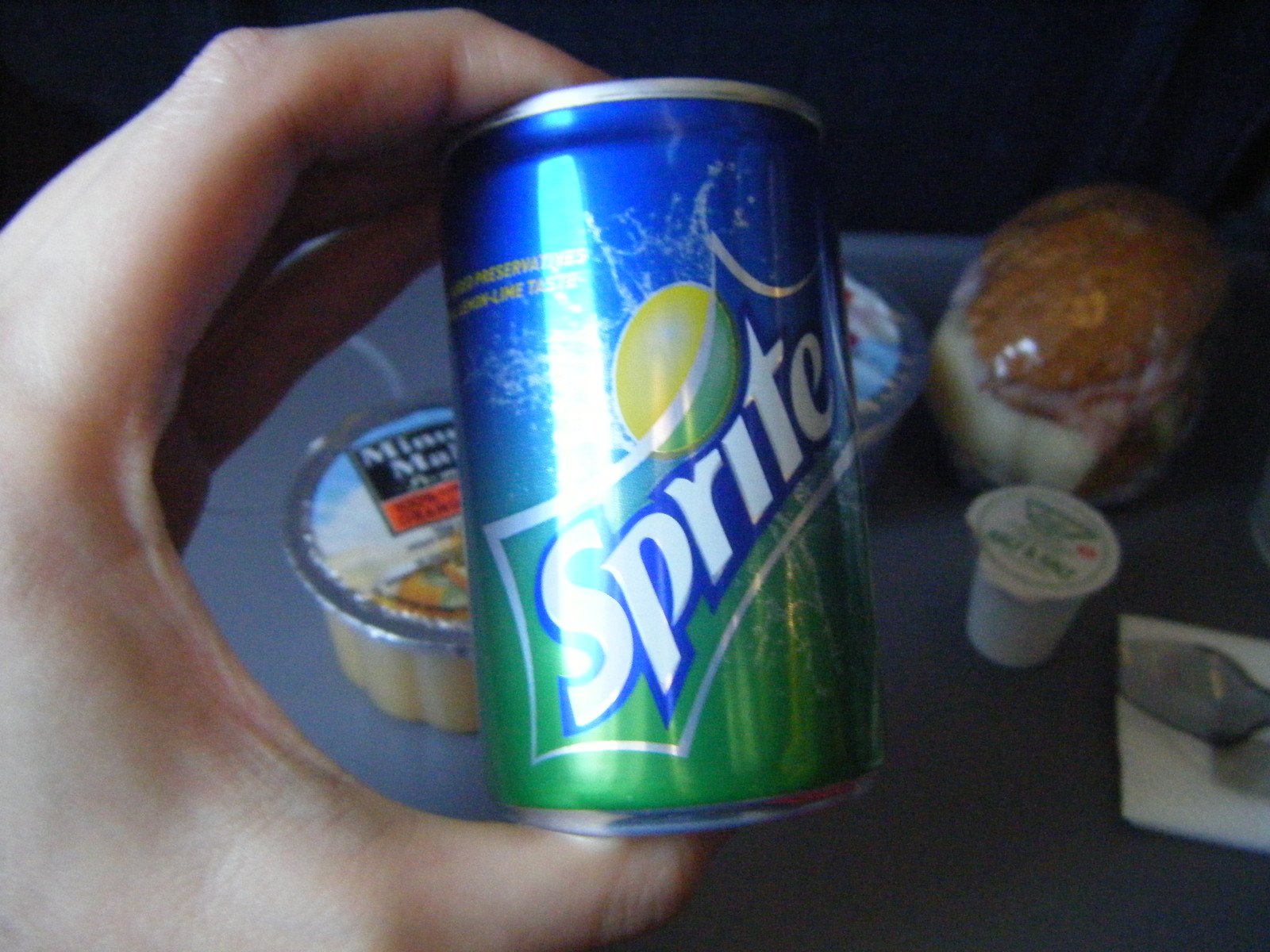In this close-up image, a hand is prominently displayed holding a mini can of Sprite. The person holds the can delicately with their index fingers positioned at the top and their thumb securing the bottom, presenting it vertically for the camera. The can itself is visually striking with a blue top transitioning to a green bottom, featuring the word “Sprite” prominently angled across the center. Just over the letter "i" in "Sprite," there is a vibrant depiction of a lemon, complemented by dynamic silver splash graphics that resemble water splashing. In the top left corner of the can, bold yellow text adds another layer of detail.

The hand holding the can is positioned over a modest gray table. In the left background, partially visible through the fingers, is a small plastic container of Minute Maid orange juice with a foil lid. Another similar container is just visible on the right side, though it is mostly hidden by the can. In the upper right corner of the image, a muffin wrapped in plastic lies on the table, while towards the bottom, a small plastic single-serving creamer is seen. In the bottom right corner, a spoon rests neatly on a napkin, adding a touch of everyday realism to the scene.